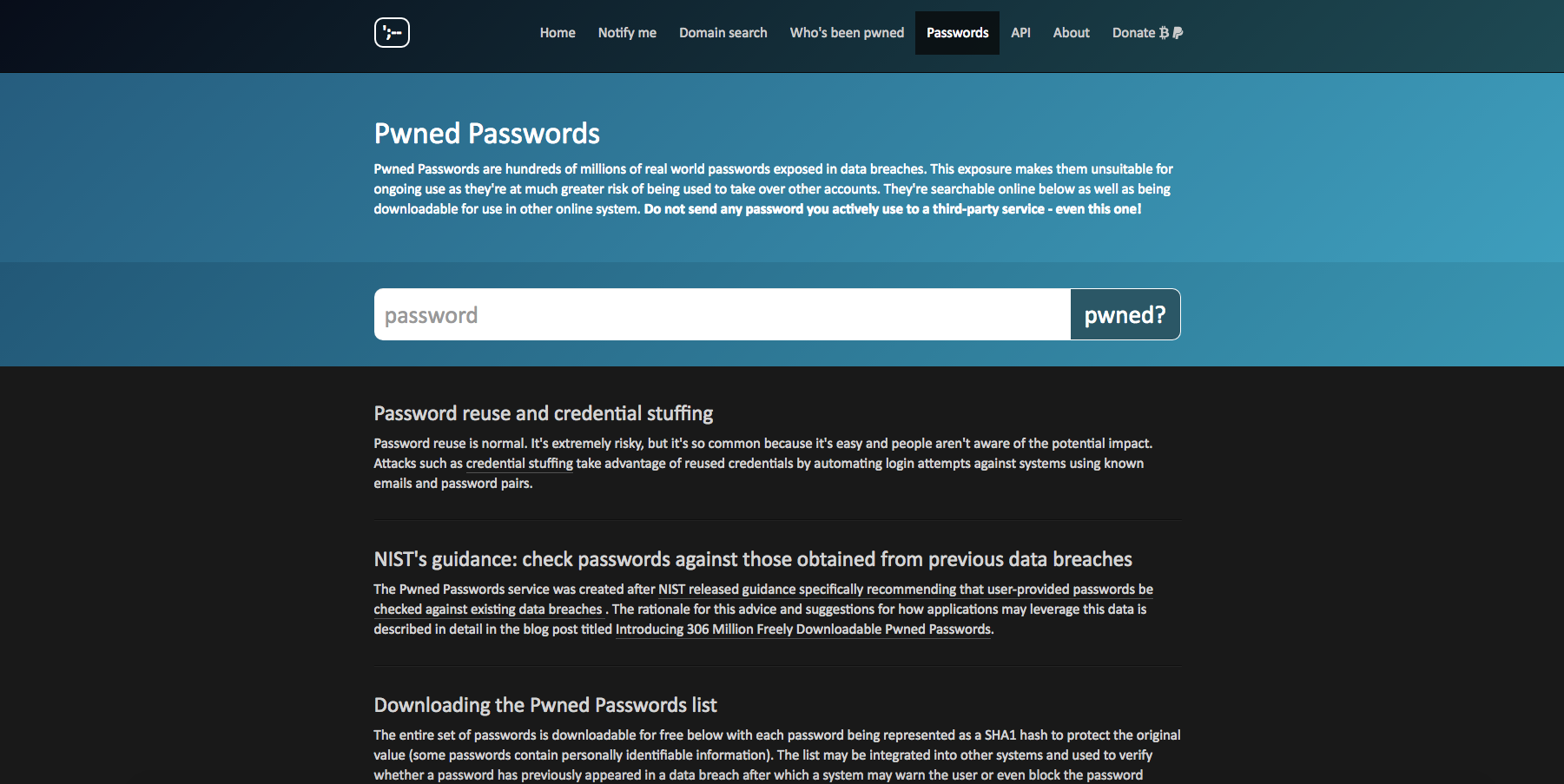The screenshot depicts a webpage with a predominantly black background. At the top of the page, there is a wide blue rectangle spanning the width of the screen, immediately followed by a slightly darker blue rectangle underneath. Within the uppermost black rectangle, a logo is situated centrally, with ample margins on both the left and right sides, creating a spacious layout. 

The text throughout the page is written in white for high contrast against the dark backdrop. At the top, in the blue section, the header "PWNED Passwords" is prominently displayed. Beneath this header lies a paragraph detailing the page's purpose.

Directly below the paragraph, within the darker blue rectangle, is a text input box presented as a white rectangle where users are prompted to type in their password. Adjacent to this input box, the text "PWNED?" followed by a question mark invites users to check the status of their password.

Further down in the black section, additional white text indicates content related to "Password Reuse and Credential Stuffing Guidance." The text provides information on checking passwords against those obtained from previous data breaches and downloading the PWNED passwords list. Each topic is accompanied by a descriptive paragraph.

Overall, the layout is clearly organized with a structured hierarchy of information, encouraging users to validate their passwords' security through a visually straightforward interface.